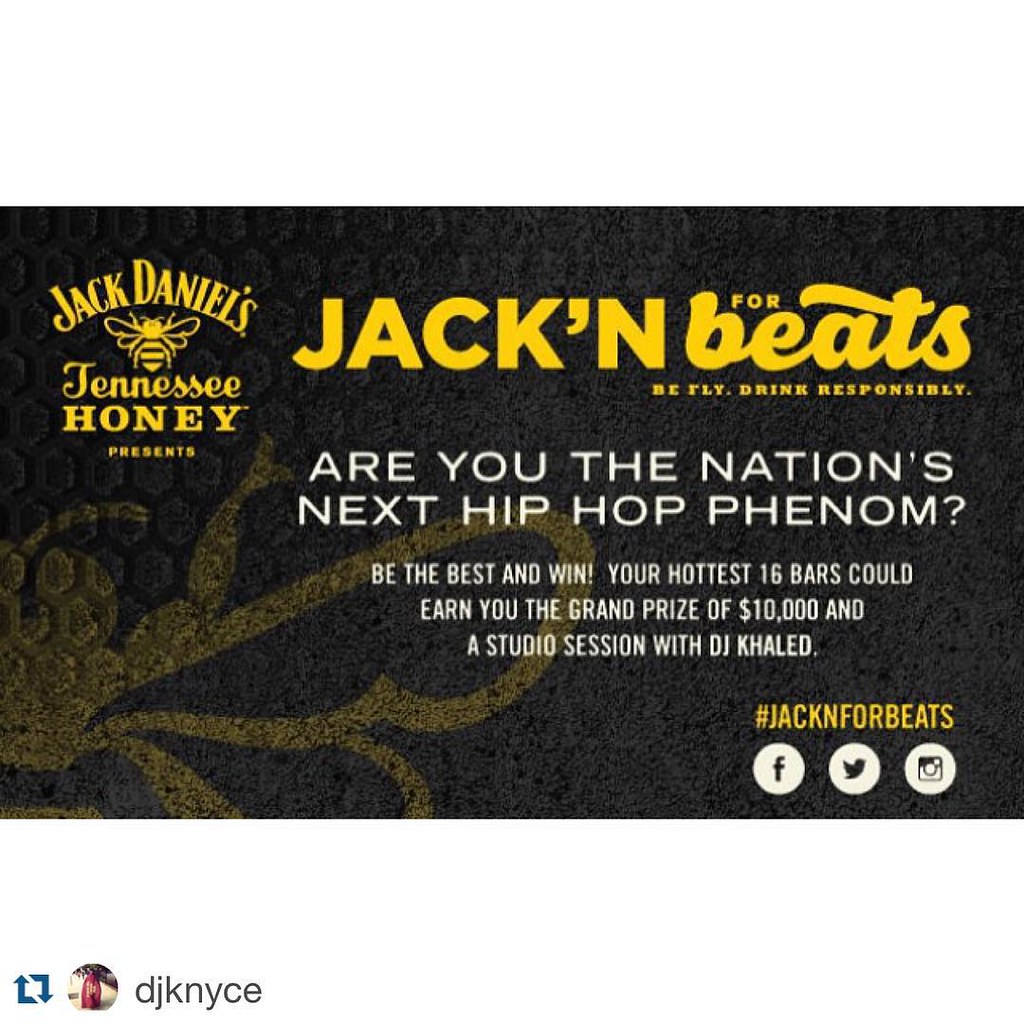The advertisement is shaped like a business card and features a black background with gold accents. In the upper left corner, the Jack Daniel's Tennessee Honey logo appears in bright yellow, accompanied by an image of a honeybee. The headline, "Jackin' for Beats," is prominently displayed across the top in yellow font, followed by the slogan "Be Fly, Drink Responsibly." Centrally positioned in white font, the text asks, "Are you the nation's next hip-hop phenom?" and encourages participants to "Be the best and win," stating that "Your hottest 16 bars could earn you the grand prize of $10,000 and a studio session with DJ Khaled." In the lower right corner, the hashtag #JackinForBeats is displayed alongside Facebook, Twitter, and Instagram icons enclosed in white circles.